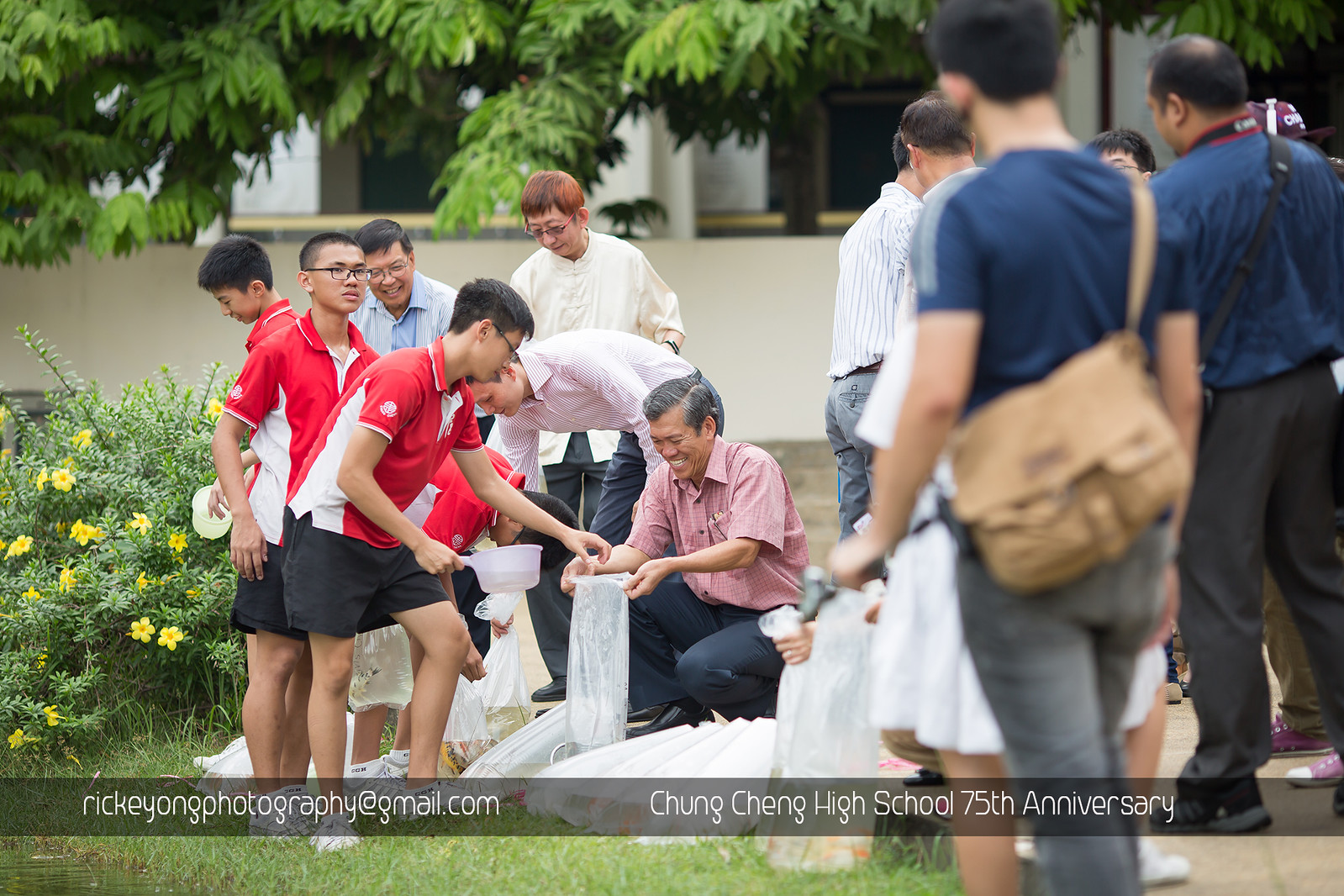In the photograph commemorating Chung Cheng High School's 75th Anniversary, a diverse group of nine to ten people, likely of Chinese descent, are gathered outdoors on a vibrant grassy area adorned with yellow flowers on the left. The background features lush tree branches and leaves, adding to the picturesque setting. Among the group are younger individuals dressed in red and white shirts and black shorts, presumably students, alongside smiling adults in various clothing, including a man in a pink shirt kneeling down in the center, holding a white bag open while a student drops something into it. Visible in the image's lower portion is a transparent black bar displaying "Ricky Young Photography at gmail.com," underlining the photograph's professional affiliation. The scene is filled with vibrant hues of blue, gray, pink, white, red, and green, capturing a moment of joyful activity and community spirit.